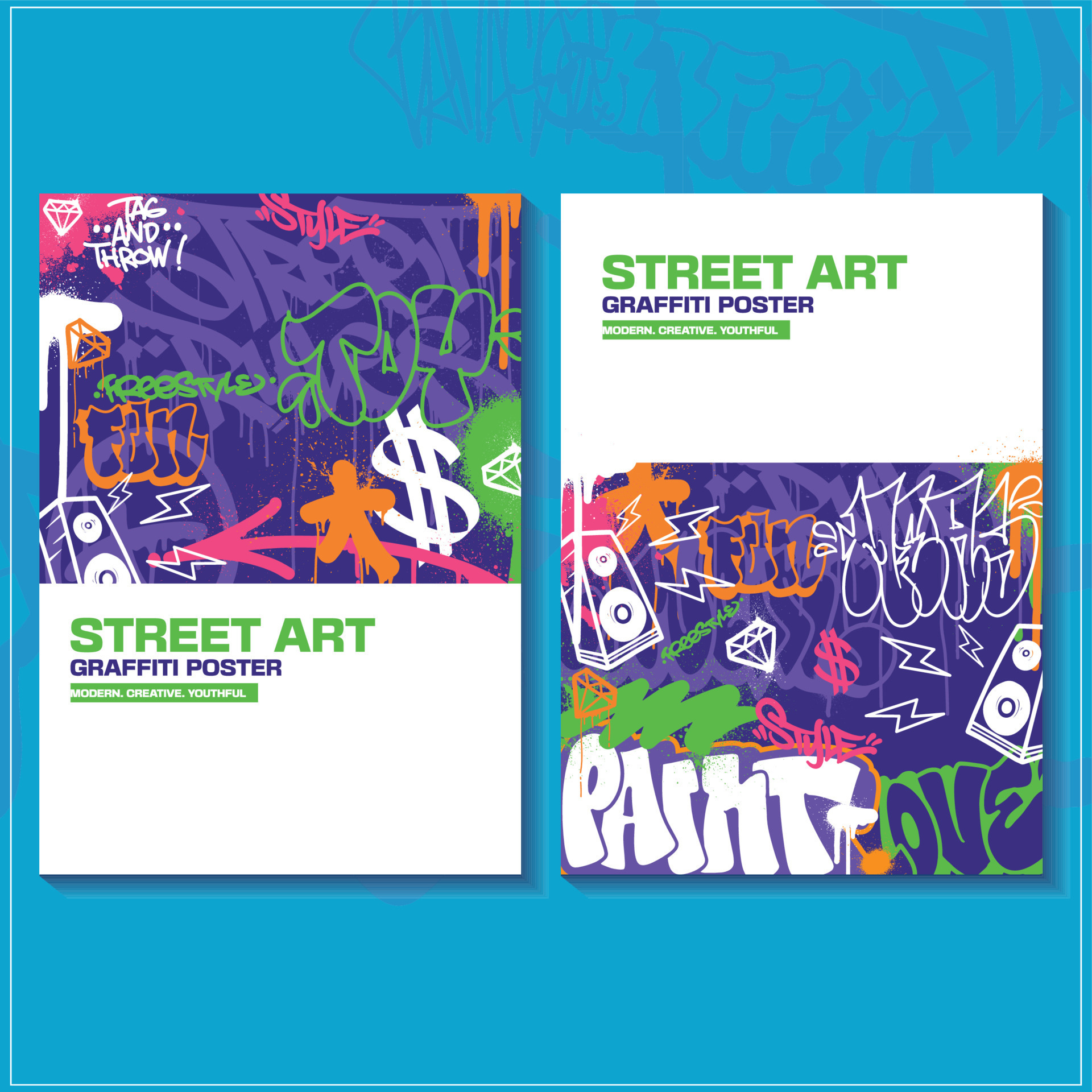This digital image comprises two adjacent street art posters on a medium blue background adorned with transparent darker blue graffiti art. Each poster features the same text— "street art, graffiti poster, modern, creative, youthful"— albeit positioned differently, creating a mirrored effect. 

The left poster displays vibrant graffiti on its upper half, characterized by a purple backdrop and a blend of white, pink, orange, and green paint. This graffiti section includes notable elements such as a white dollar sign, green bubble letters spelling "toy," and white letters that say "tag" and "throw" alongside white and orange diamonds with speakers emitting lightning bolts. The bottom half contains a plain white box with the aforementioned text.

Conversely, the right poster has this white boxed text at the top, switching places with the graffiti artwork, which occupies the lower half. The entire image thus creates a visually compelling interplay of text and graffiti art, set against its blue background.